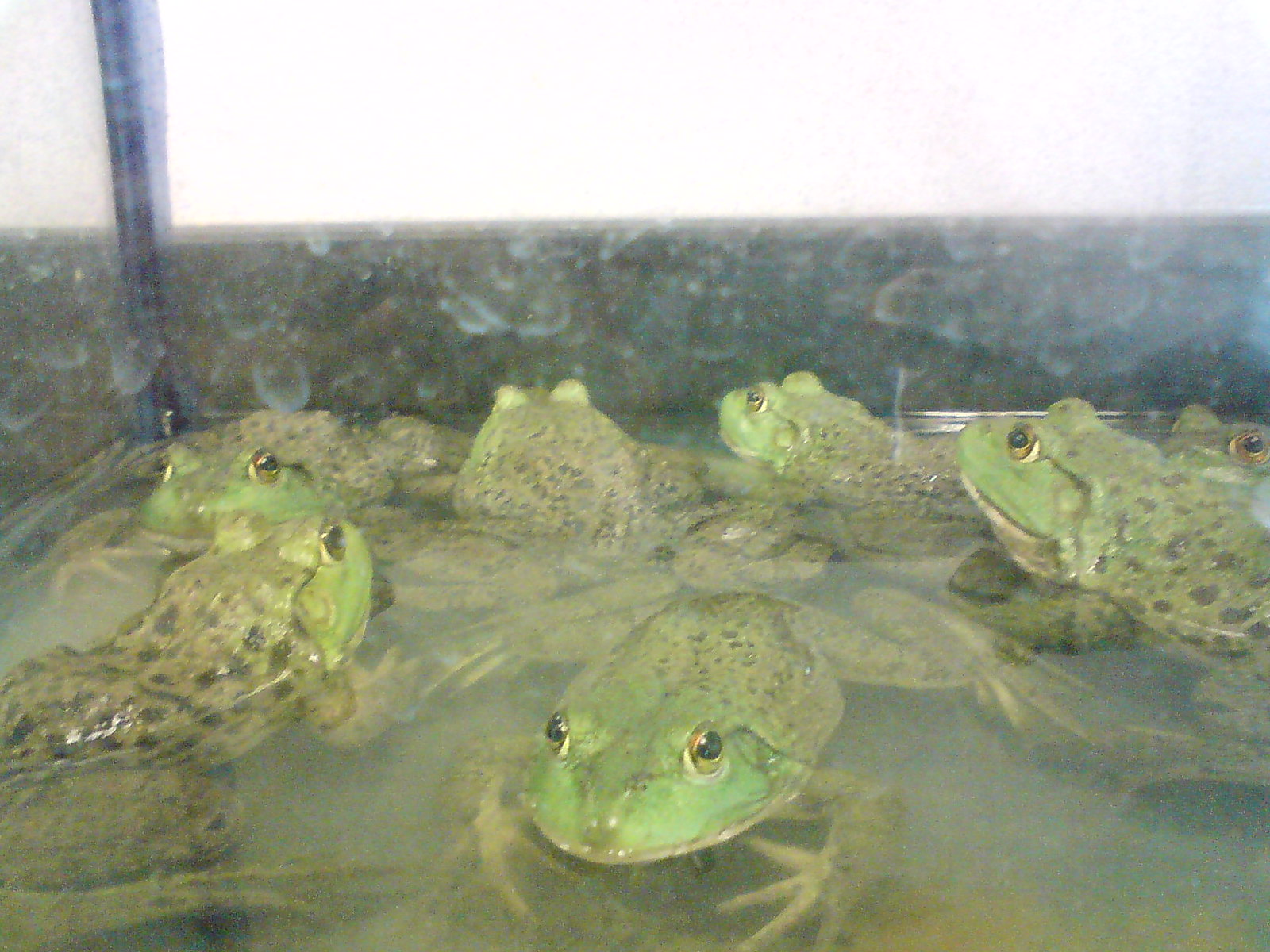This image features a small glass aquarium, or terrarium, showcasing seven green frogs in a shallow pool of water at the bottom. The frogs have distinctive dark green bodies speckled with black and brown freckles, with solid green snouts and light green, elongated fingers. Each frog has two prominent lumps on their heads where their black, beady eyes are located. The backdrop of the aquarium includes a top white wall, green marble siding, and a blue partition on the right. The blue pillar also appears on the left side. The glass is slightly blurred, suggesting it might be unclean, but the vibrant details of the frogs and their habitat are still visible. Some frogs are fully submerged, displaying their speckled bodies, while others have their bright green faces peeking out of the water.